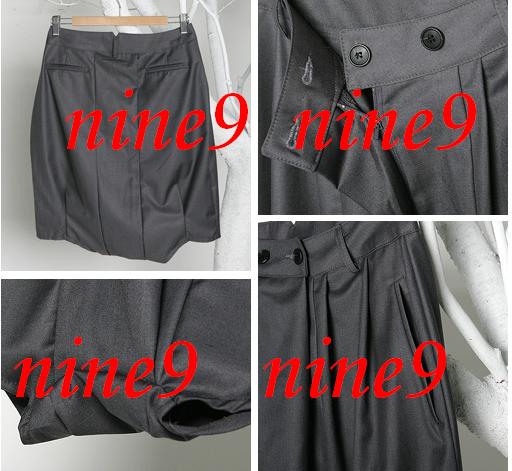The composite image features a series of four photographs, showcasing a unique dark gray garment that appears to be a fusion between a skirt and shorts. The main highlights of the piece include a built-in waistband and two side pockets positioned at the top, one on the left and one on the right. Each photo gives a distinct perspective of the garment's details: 

1. The first image displays the entire outfit hanging on a metal hanger with a wooden grip, against a white background. In bold red text, the word "nine" is written out, followed by the numeral "9".
2. The second image offers a close-up of the waistband, emphasizing the two-button configuration—one gray and one black, each with two holes.
3. The third image captures the lower part of the garment, revealing how it slightly angles at the bottom to form an almost trapezoidal shape.
4. The final image zooms in on the upper right section, maintaining the same text in a red font against the white backdrop.

Throughout all four images, the brand name "nine9" is consistently printed in red, reinforcing the garment's identity.